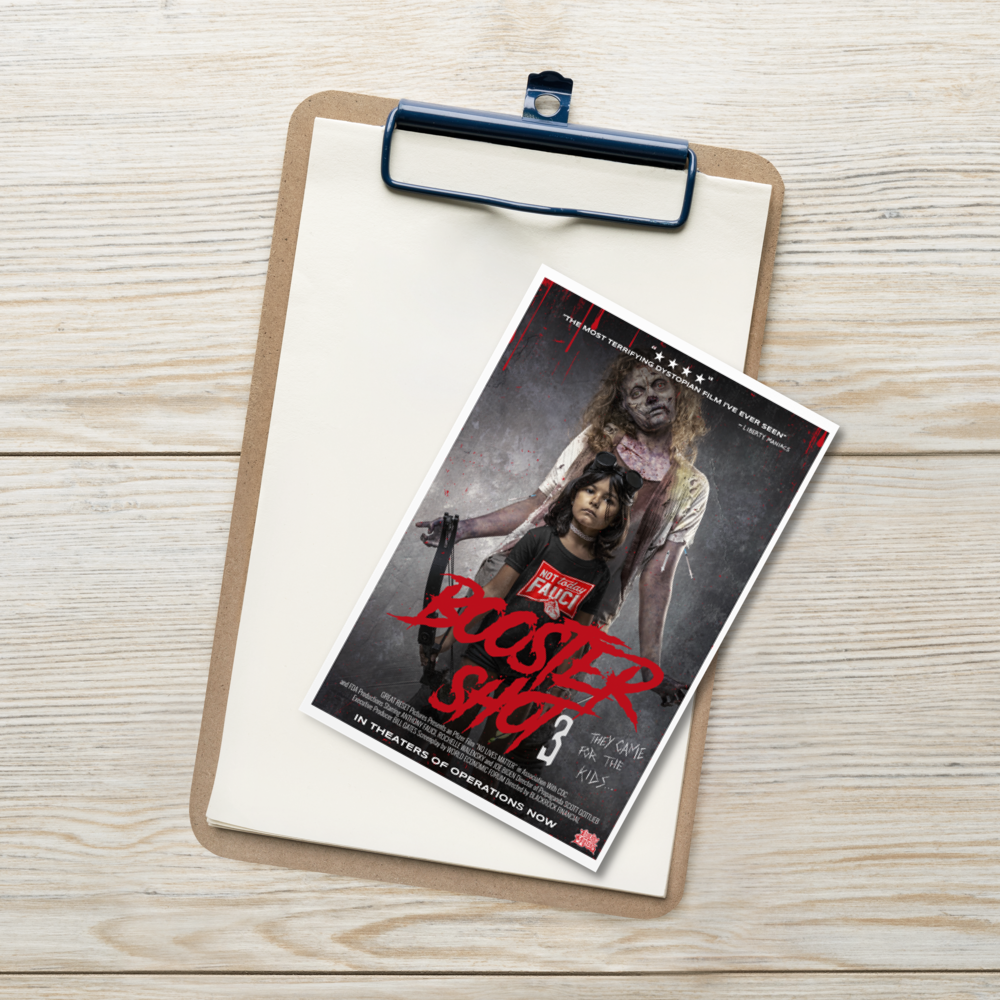The image features a close-up of a setup with a light-colored, almost white wood table as the background. On top of the table is a darker wood clipboard with a black metal clip, holding a standard size, white, blank sheet of paper. Overlaid on the paper is a tilted movie poster promoting "Booster Shot 3." The poster, rendered with a graphic design aesthetic, depicts a gruesome zombie character with long hair, a grayish complexion, wearing a short-sleeved, brown tank top and white shirt, standing with arms outstretched and head cocked to the right. In front of the zombie stands a young girl, approximately six or seven years old, with dark hair, a dark top (possibly emblazoned with the word "Fauci"), a choker necklace, and goggles perched on her head. The title "Booster Shot 3" is written at the bottom of the poster in a blood-soaked red font, with the number '3' in plain white. Below that, white text reads, "In Theaters of Operations Now."